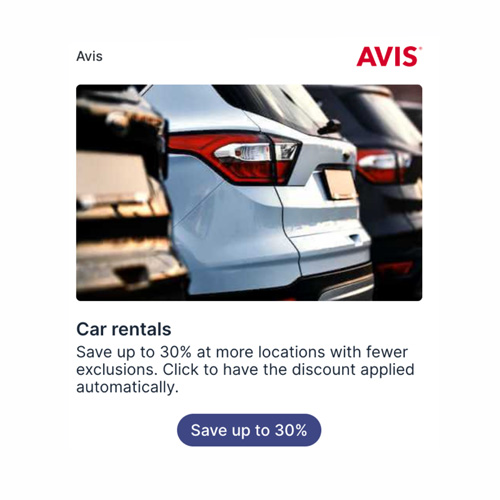A promotional screenshot showcases three SUVs in brown, white, and black colors. The image prominently features the Avis logo in red, emphasizing their car rental services. The text highlights a special offer: "Save up to 30% at more locations with fewer exclusions." Additionally, there's a purple oval with white text that reiterates the "Save up to 30%" discount, which can be applied automatically by clicking.